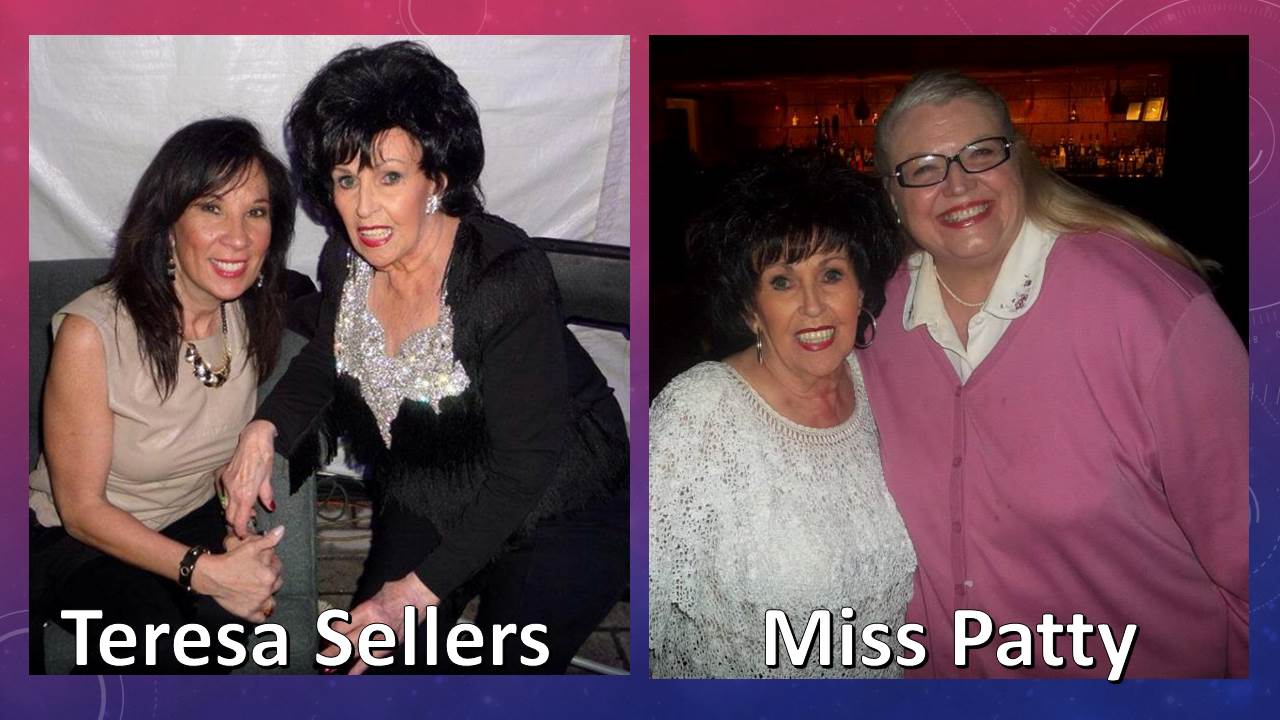In this image, there are two side-by-side photographs set against a backdrop of various shades of purple. The left photograph features two women seated close to each other, labeled "Teresa Sellers" in white letters below the image. The woman on the left is adorned with black hair, styled in a large hairdo, a light brown blouse, black pants or skirt, and accessorized with a white and black necklace, earrings, and lipstick. The woman on the right in this photograph wears a black blouse with a silver scoop neck and black pants, also with black hair. Both appear to be leaning towards each other in a seemingly intimate pose.

The right photograph captures two women standing side by side, labeled "Miss Patty" in white letters beneath. The woman on the left wears a white ruffled dress, dark hair, red lipstick, and earrings. The woman beside her on the right is a larger figure with blonde hair, dark glasses, a pink sweater over a collared white shirt, and adorned with red lipstick. The background of this photograph appears to be a dimly lit room with no discernible details. The image is framed with a red and blue border, completing the detailed presentation of these portraits.